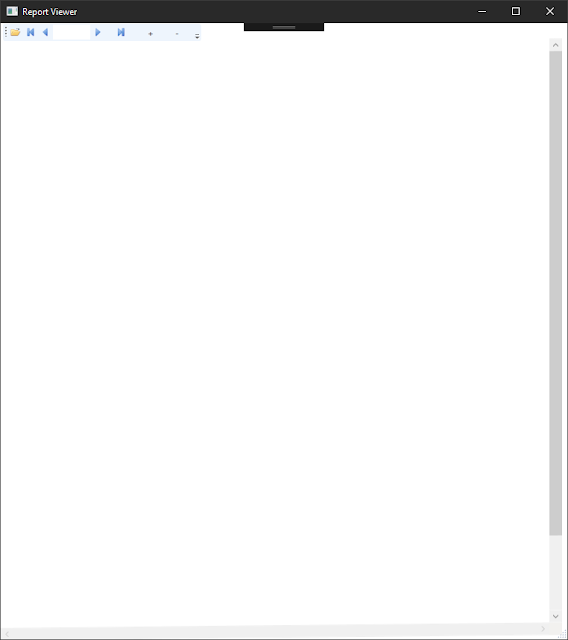The image is a vertically rectangular screenshot of a report viewer interface. At the top, there is a thin black horizontal banner featuring a report icon on the upper left, followed by the white text "Report Viewer." On the upper right of the banner, there are the minimize, expand, and close window icons. Below this banner, the left side of the interface hosts a series of functional buttons, including a file icon, back navigation icons, and an open white space. Extending towards the right, there are right directional icons, a plus icon, and another indistinctively small icon that looks like it might be a minus symbol. The majority of the image showcases a blank, white page resembling a document or report with no text or content displayed. Additionally, on the right edge of the interface, there is a vertical scroll bar for navigating up and down, and at the bottom, there is a horizontal scroll bar for side-to-side navigation.